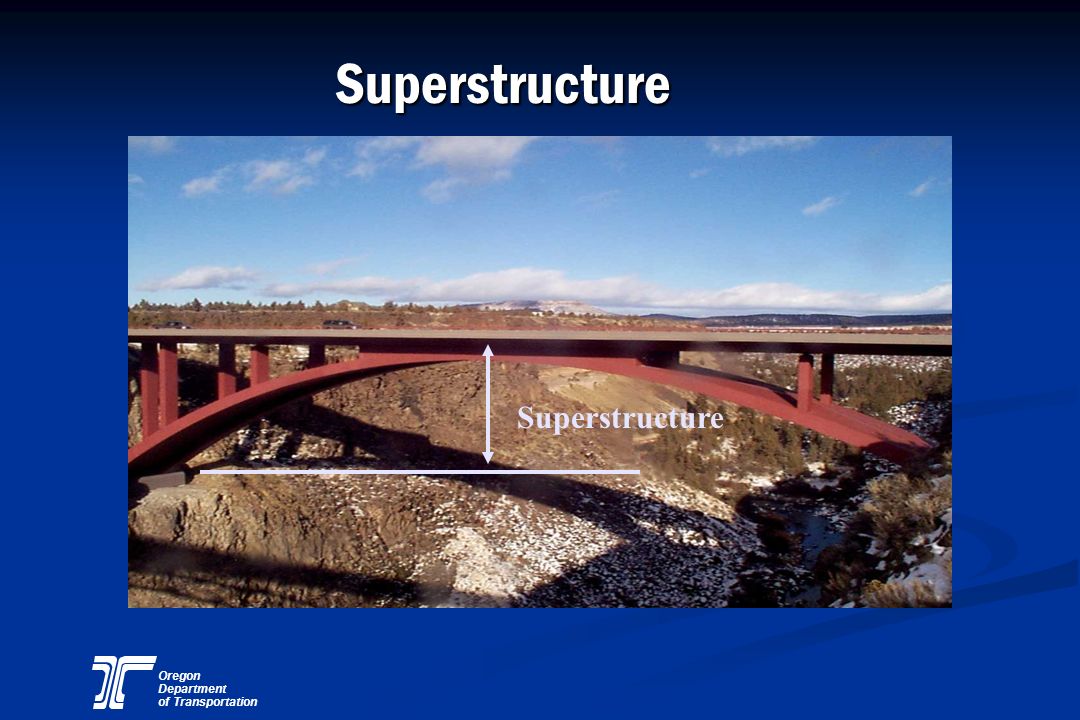The image presents a detailed depiction of a red steel girder bridge spanning from one side of a canyon to the other, prominently positioned in the center of the photo. The bridge, located over a rugged landscape featuring dirt hills, brown rocks, patches of green grass, and scattered snow, is captured with clarity, extending horizontally across the scene. Above the bridge, the sky is illustrated with shades of blue and interspersed white clouds. At the top of the image, bold white text reads "Superstructure," echoed by a similar label directly on the bridge with an arrow pointing vertically, further emphasizing this architectural element. The image appears as part of an information slide, with a blue gradient background that darkens towards the top and features a subtle swirl pattern at the bottom right. The slide, possibly from a company presentation, includes the Oregon Department of Transportation logo and name in white text located at the bottom left corner. The composition and layout suggest a professional setting aimed at providing detailed information about the bridge's superstructure.